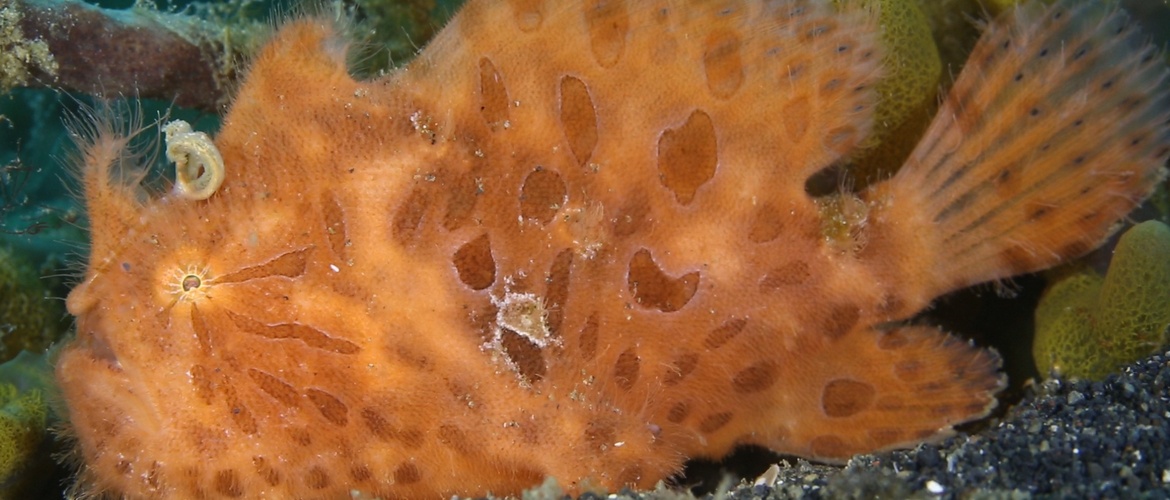The photograph captures a close-up of a peculiar deep-sea fish, primarily orange with darker orange and red cat-like spots reminiscent of a cheetah pattern. The fish features strikingly unusual green-blue eyes, and a sensory appendage adorned with hair-like fibers extends from its nose, protruding several inches. Around its head and possibly across its entire body, a fuzz-like texture is visible. Below one of its eyes, there are markings that give an impression of sunlight rays, enhancing the fish's exotic look. The image's background reveals an underwater scene with light blue hues, coral, algae, and rocks, suggesting either an aquarium or a natural ocean floor setting. The fish's tail and fins, also covered in spots, are clearly detailed. There's a white object on the fish, which could either be part of the fish or an external parasite. The detailed plumage near its mouth and additional fin behind the visible eye add to the complexity and beauty of this intriguing underwater creature.